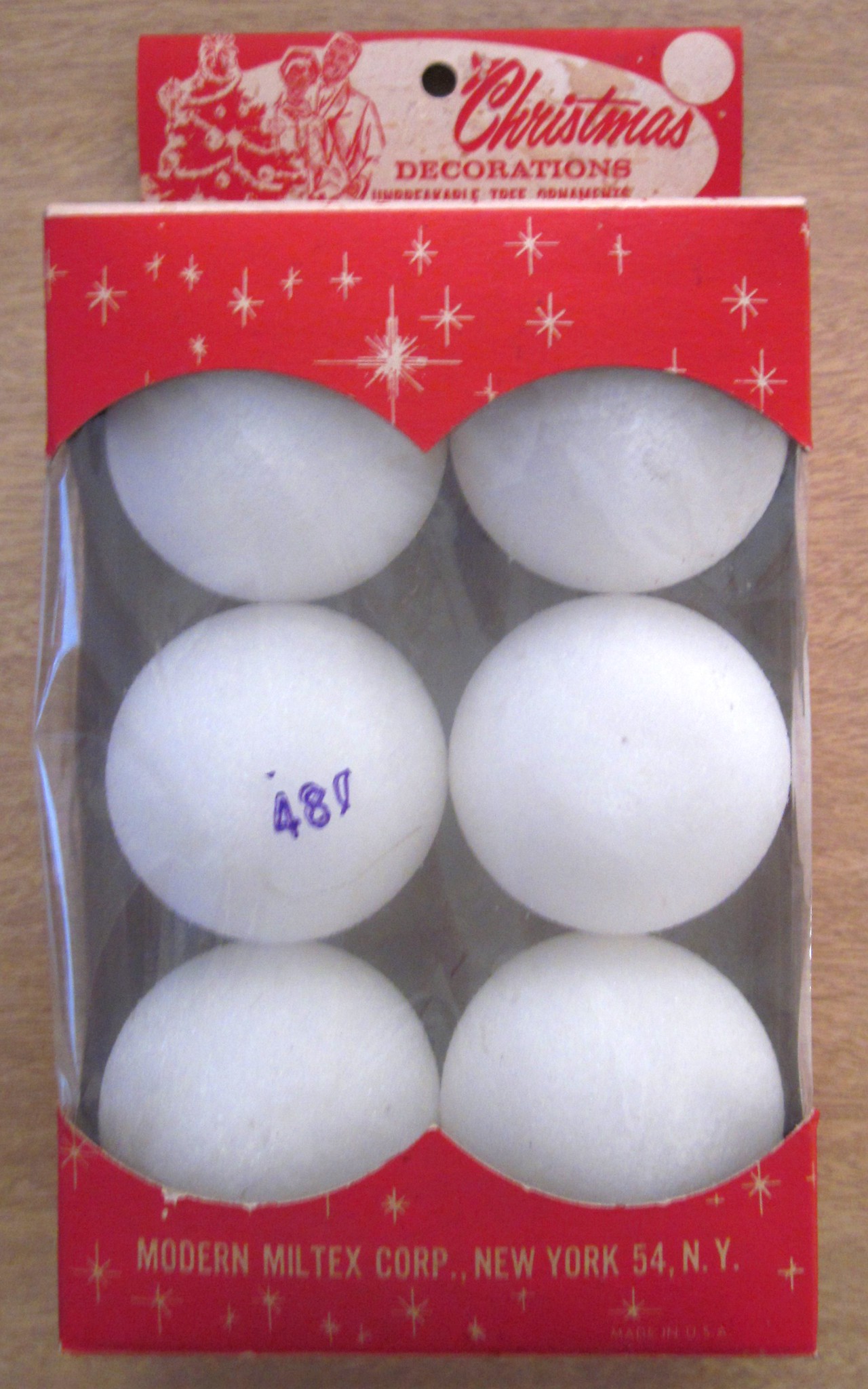The image is a color photograph in portrait orientation featuring a vintage package of Christmas decorations. The packaging, which occupies most of the frame, is predominantly red and white with various festive graphics and text. At the top of the packaging, the text "Christmas Decorations" is displayed, with "Christmas" in a decorative red font. Below this text, though partially blurred, is another line that cannot be discerned. The top-left section of the cardboard hanger has a hole punched for displaying the package on a store rail.

The design includes a red and white illustration of an elderly 1950s-style couple standing beside a Christmas tree adorned with tinsel and ornaments. The entire pattern of the box is festive with decorative stars. The central part of the packaging features a clear cellophane window through which six white bulbs are visible, one of which has a blue stamp reading "48."

At the bottom of the packaging, another section of cardboard reinforces the cellophane window and displays the manufacturer's information: "Modern Miltex Corp, New York 54, N.Y." The box rests on a light brown, wood-like surface, enhancing its vintage appearance.